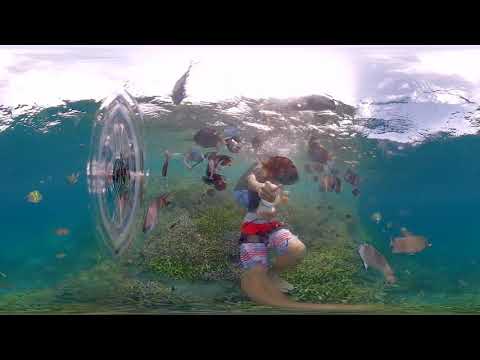The image is a wide rectangular photograph capturing a distorted underwater scene framed by thick black bars at the top and bottom. The water, which makes up the majority of the image, is a bright turquoise blue. At the center appears to be a reflective glass or plastic object with a person partially visible, their hand extended toward the lens. The person's features are blurred, but they seem to be wearing blue and red shorts. A small yellow fish swims to the left of the central object, while two large gray fish hover near some greenery that the person appears to be sitting on. The sky above is visible, filled with light gray and white clouds, indicating a daytime setting. The distortions, possibly from a lens effect, give the impression of viewing through a tank or aquarium, enhancing the surreal underwater tableau.